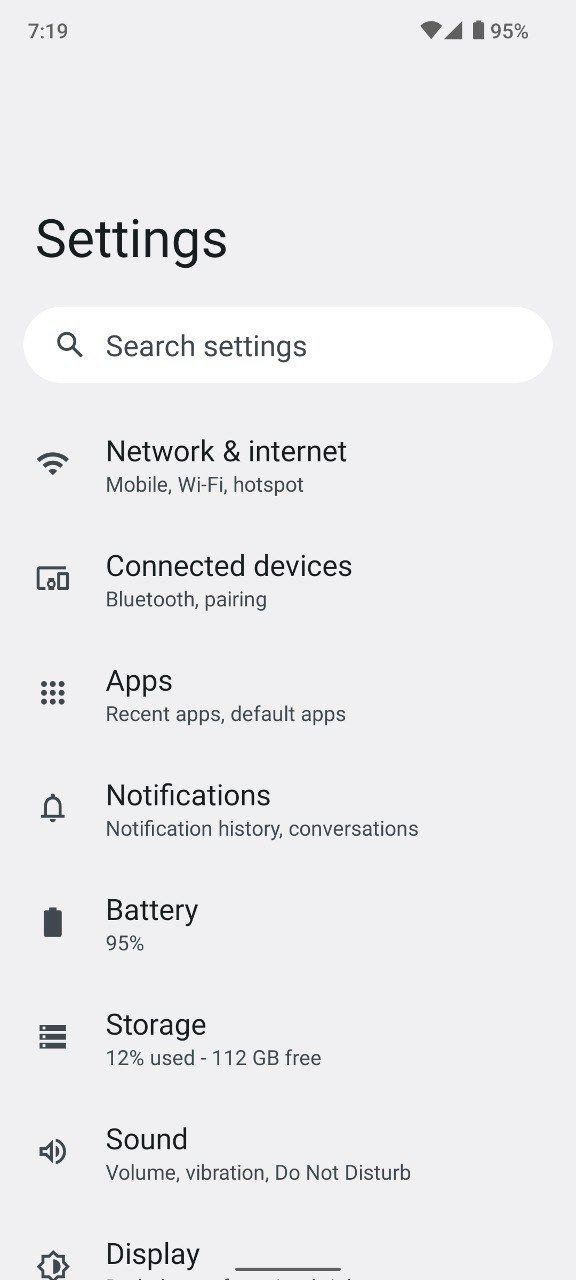Screenshot of a smartphone settings menu displayed at 7:19 AM, as indicated by the clock at the upper left. The status bar shows full Wi-Fi signal, full cellular signal, and a battery level of 95%. The title "Settings" is prominently shown in large black text.

The menu lists nine options, each accompanied by an icon on the left:

1. **Search Settings**: Represented by a magnifying glass icon.
2. **Network & Internet**: Depicted with a Wi-Fi beacon icon. This option likely includes settings for Wi-Fi, mobile data, and hotspots.
3. **Connected Devices**: Shown with an icon of a screen, phone, and watch, indicating settings for Bluetooth pairing and connected devices.
4. **Apps**: Represented by a grid of nine dots, with options for recent apps and default apps.
5. **Notifications**: Illustrated with a bell icon, providing access to notification history and conversations.
6. **Battery**: Indicated by a battery icon, showing 95% battery life.
7. **Storage**: Shown with an icon resembling three server racks, indicating 12% used and 112 GB free.
8. **Sound**: Represented by a speaker with sound waves, offering options for volume, vibration, and Do Not Disturb.
9. **Display**: Depicted with a sun icon; however, the detailed options under 'Display' are not fully visible in the screenshot.

The background is a shade close to white but not pure white, with slight discoloration noticeable.